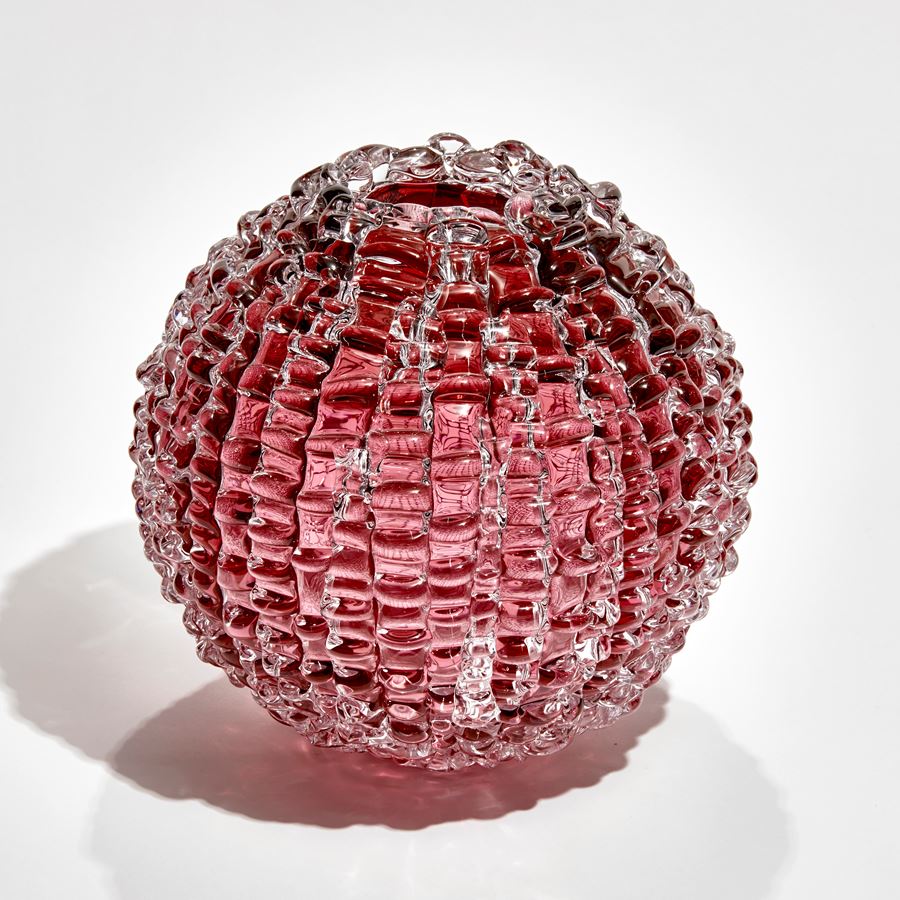The image depicts a striking glass sphere set against a pristine white background. The sphere features a unique, heavily textured exterior resembling drippy, bumpy glass or pebbled ice, creating a fascinating, tactile appearance. Through the clear glass, a deep, dark red substance is visible, adding a rich, colorful contrast to the transparent outer layer. There is an apparent hole at the top of the sphere, where this red color seems to have been introduced. The sphere casts two distinct shadows due to the overhead lighting—a darker, more pronounced shadow to the left and a lighter one directly beneath it. The object, which might be mistaken for an intricate piece of jewelry or a decorative bead, enhances the overall allure with its reflective and shiny surface, capturing any light that hits it beautifully.